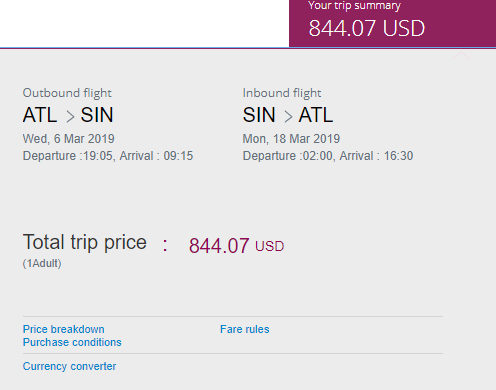A detailed caption for the given image could be:

"This cropped screenshot showcases a section of an airline booking page, specifically the trip summary and cost details. In the top right corner, a small purple box prominently displays 'Your Trip Summary' in white text, with the total trip cost of $844.07 USD in large numbers underneath. Below this, a large gray box outlines the flight details. On the left side, it specifies 'Outbound Flight: Atlanta to SIN,' and on the right, it reads 'Return Flight: SIN to ATL.' The total trip price is reiterated as $844.07 USD. At the bottom left, it indicates 'One Adult.' Further down, in blue font, clickable options for 'Price Breakdown,' 'Purchase Conditions,' 'Fare Rules,' and 'Currency Converter' are listed. The departure and arrival dates and times for each flight segment are also detailed under their respective headings. A dark purple bar adorns the top edge of the screenshot, framing the information provided."